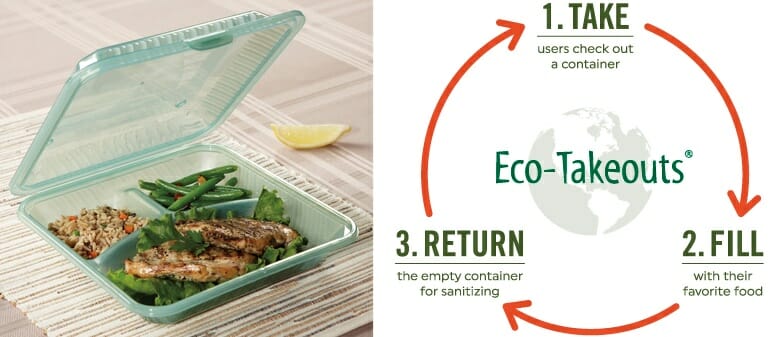The image is an advertisement and set of instructions for using the "ECHO-takeouts" eco-friendly food container system. The ad is visually divided into two parts. On the right side, a circular instructional graphic features prominently. The circle is segmented into three parts, each annotated with a red arrow guiding through the process. Starting at the top with "1. Take," users are instructed to check out a container. The arrow then moves to the 4 o'clock position with "2. Fill," showing users filling the container with their favorite food. The sequence concludes at the 7 o'clock position with "3. Return," where users are instructed to return the empty container for sanitizing. At the center of this circle, the words "ECHO-takeouts" are displayed over a transparent globe, reinforcing the eco-friendly theme.

On the left side of the image, there is a clear example of the food tray in use. The take-home container, made of pale green plastic with a faint tint, has both a top and bottom part, although the top is currently open and connected to the lower portion. This container is divided into three sections: the largest section contains grilled chicken breast pieces placed on lettuce leaves, the top left section holds rice mixed with vegetables, and the top right section contains green beans. A lemon wedge is placed to the side of the tray on a gray, plaid-patterned placemat featuring alternating vertical stripes. The overall setup shows the container slightly tilted to the right, providing a comprehensive view of the food arranged within.